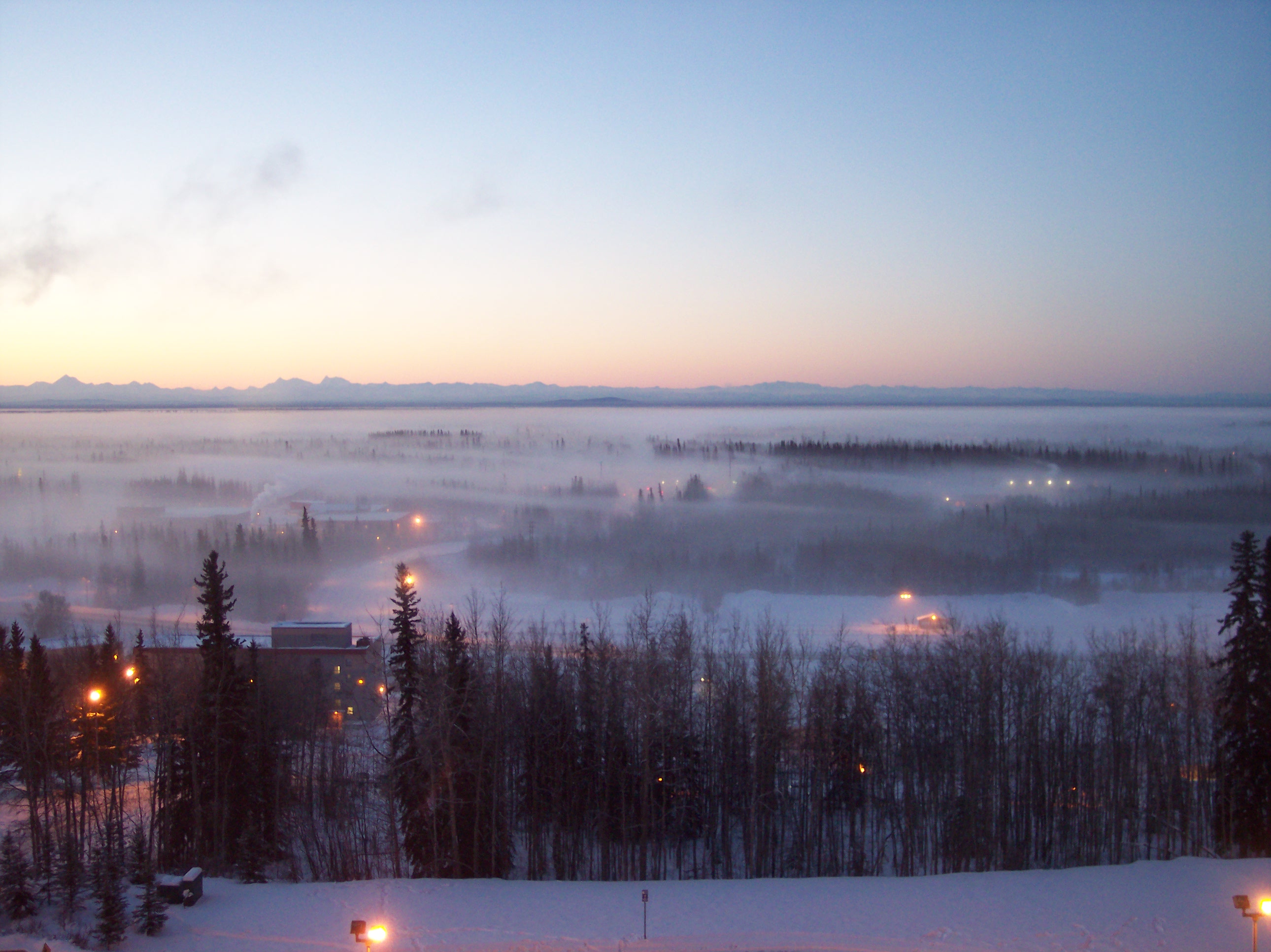This is an aerial photograph of an extensive, snowy winter landscape at twilight, just after sunset. The sky in the distance still retains a hint of light, with hues ranging from steel grays to blues and a faint haze of amber along the horizon. Below, untouched snow blankets the ground, stretching across a vast area interspersed with clusters of tall, thin trees and small building structures, their lights casting amber halos in the misty atmosphere. A dark tree line silhouettes against the fading evening light, cutting horizontally through the center of the image. The landscape features several little peninsulas jutting into a visible river or large body of water, which reflects the dimming sky. On the left side of the photo, a roadway snakes from the lower left corner toward the center, flanked sporadically by buildings illuminated with yellow lights. Additional floodlights and spotlights cast subtle glows on the snow-covered ground, while in the distance, the smoky outline of more trees and buildings fades into the foggy horizon.